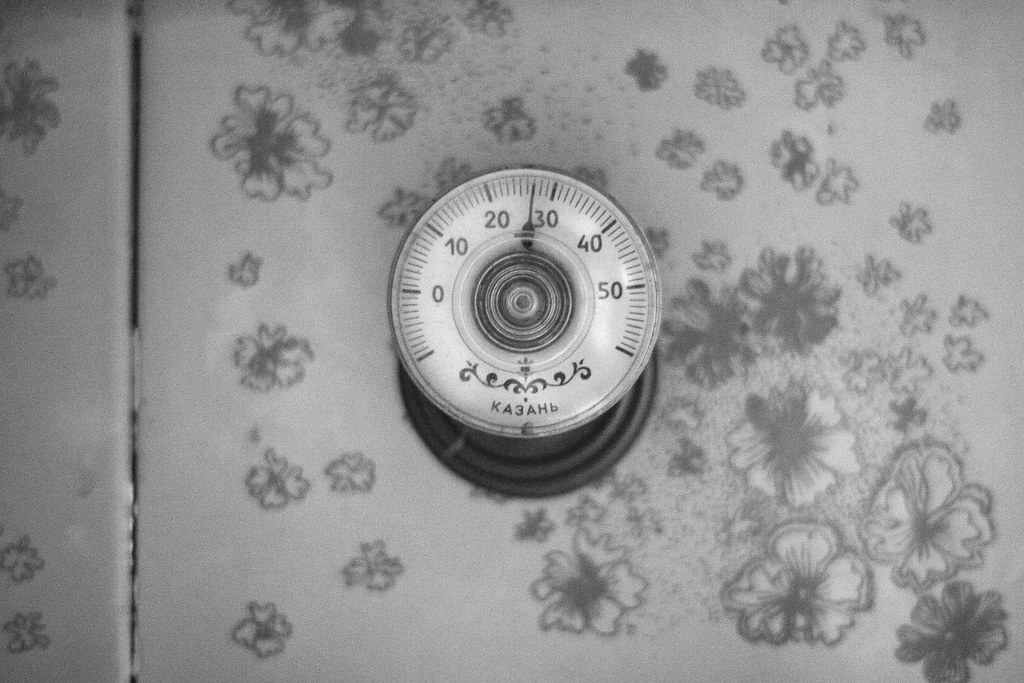This is a black and white photograph featuring a circular gauge mounted on a wall adorned with a floral pattern. The gauge is positioned centrally, partially obscuring another circular object behind it that contains three smaller black circles. The gauge itself is marked with numerous lines along its circumference, with thicker lines denoting increments of ten. The numbers visible on the gauge are 0, 10, 20, 30, 40, and 50. A needle on the gauge points between the 20 and 30 marks, closer to 30. Below the numerals, the gauge is embellished with a floral decoration echoing the wall's pattern. To the left side of the image, a pronounced black line divides the composition, suggesting the presence of a border or seam on the tiled wall. Additionally, there are inscriptions in Cyrillic script visible on the lower part of the gauge.